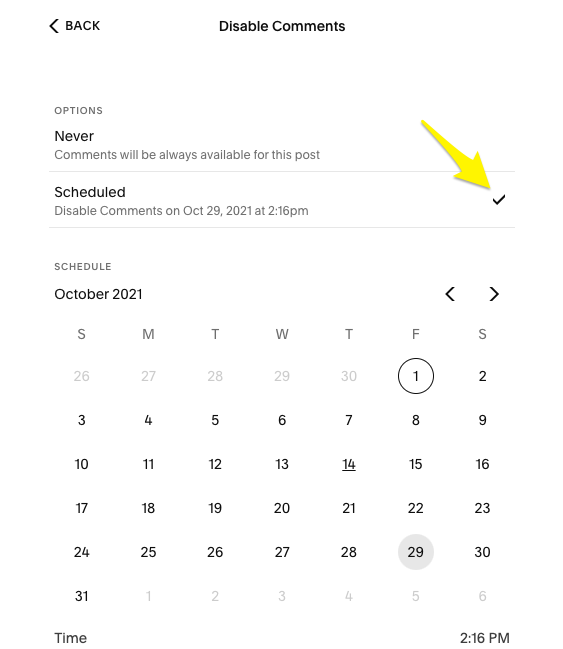This image is a detailed screenshot of a calendar interface designed to disable comments on a post. At the top of the image, the phrase "Disable Comments" is displayed in bold black text, alongside a black back button for navigation. Below, there are two options for comment settings: "Never," which ensures comments stay available indefinitely, and "Scheduled," which indicates disabling comments on October 29, 2021, at 2:16 PM. A black check mark is visibly selected next to the "Scheduled" option. A prominent yellow arrow points directly at this check mark, highlighting the selection process for disabling comments, suggesting that this image is used for instructional purposes. The calendar displayed shows the month of October 2021, with specific scheduling options. Notably, October 29, the day marked in the schedule, is one day before the user's girlfriend's birthday.